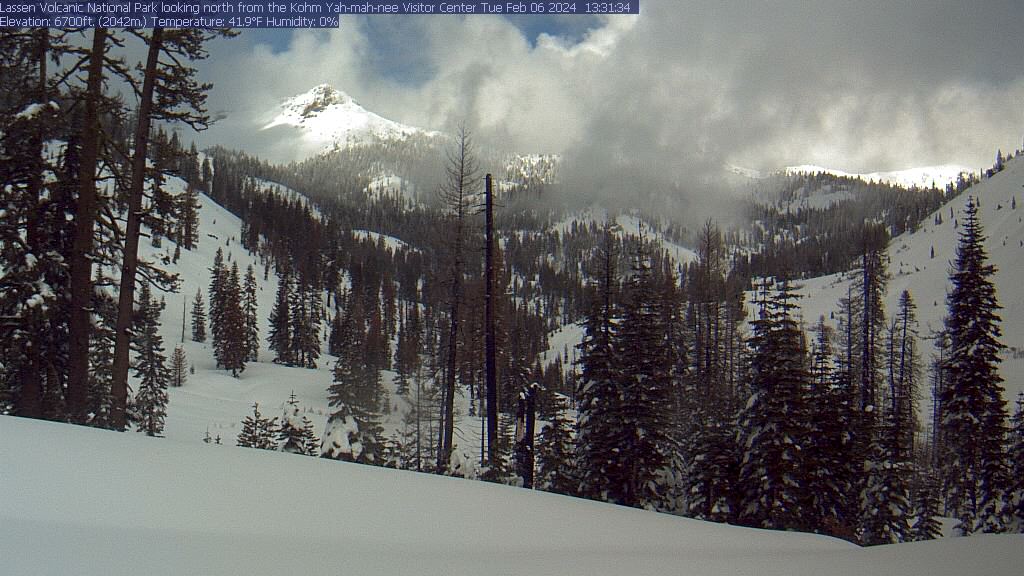This image is a detailed, color photograph taken outside, presumably by a scientific camera, capturing the serene and crisp beauty of Lassen Volcanic National Park. Looking north from the Qom Yamani Visitor Center on Tuesday, February 6, 2024, at an elevation of 6,700 feet (or 2,042 meters), the temperature is noted at 41.9 degrees Fahrenheit with 0% humidity.

The scene unfolds under a bright, blue sky dotted with scattered white clouds, giving a vibrant backdrop to the winter landscape. In the foreground, the snow-laden ground contrasts vividly with a cluster of Christmas trees standing tall, their branches draped in delicate layers of snow. Dominating the middle ground is a peculiar pole that could be a burnt tree, adding a touch of mystery to the image.

Beyond these trees, the mountainous terrain rises, with peaks and valleys generously covered in snow. Evergreen pine trees stretch up the mountainside, their needles catching the light snow. In the distance, a colossal, snowy mountain peak stands tall, partially illuminated by sunlight while the rolling clouds weave through the valleys, creating pockets of shadow that add depth and drama to the scene. The timestamp on the image reads 13:31.34, marking a moment in this picturesque winter day. 

This stunning photograph meticulously captures the tranquility and majesty of the Alaskan wilderness on a winter day, immortalizing the ethereal beauty of nature in precise detail.